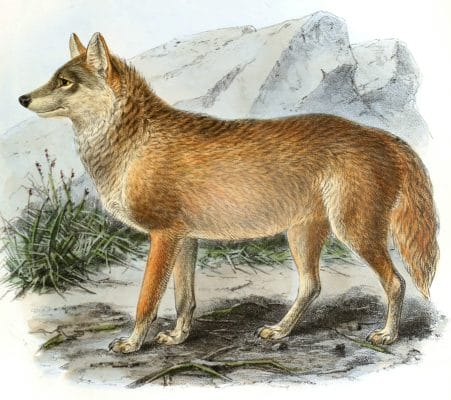This is a detailed, hand-drawn colored illustration, likely from an 1800s or 1900s field guide, featuring a coyote. The side view of the animal captures its mid-step stance as it looks to the left with its pointed ears up, appearing to listen intently. The coyote's coat is a striking mix of orangish-red tones with tannish hues, complemented by grayish facial markings, a black nose, thick tail, and whitish paws. The natural environment surrounding the coyote includes a gray and brown ground, dotted with twigs, roots, and small patches of green grass. Behind the coyote, a rugged mountain range with white and gray rocky peaks looms, emphasizing the wild and untamed setting. The illustration's meticulous detail and coloration suggest it serves as an educational depiction within a collection of wildlife illustrations.